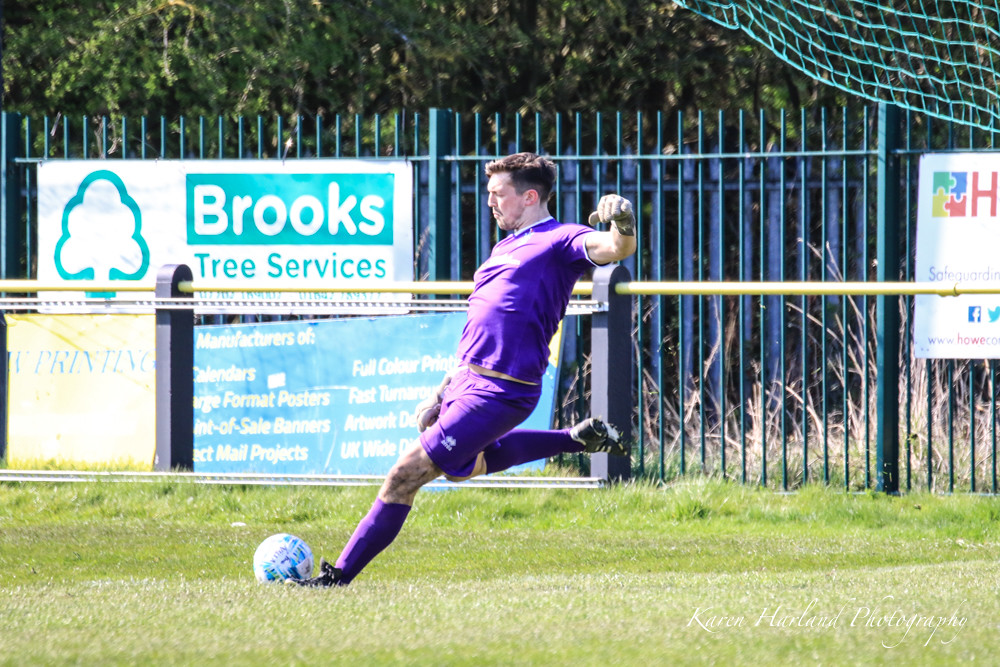In this dynamic outdoor photograph, a soccer player, outfitted in a purple uniform complete with matching top, shorts, socks, and gloves, is captured mid-motion as he prepares to kick a stationary soccer ball. He exudes concentration, with his body leaning back and leg extended in readiness. The player has brown hair and sports a bit of a mustache and beard.

The green grass beneath him appears well-maintained, with patches reflecting a silvery shimmer under the sunlight. In the background, a metal fence adorned with sponsor banners stands out. A prominent turquoise banner advertises Brooks Tree Services, positioned to the left of the image. Beneath it, another banner, in a combination of yellow and blue, promotes "Full color prints, fast turnaround." Adjacent to these, a white banner with text including "safeguard" and icons for Facebook and Twitter can be seen, along with a hint of another ad featuring blue netting. Beyond the fence, a line of trees and some bushes provide a natural backdrop to this small stadium scene.